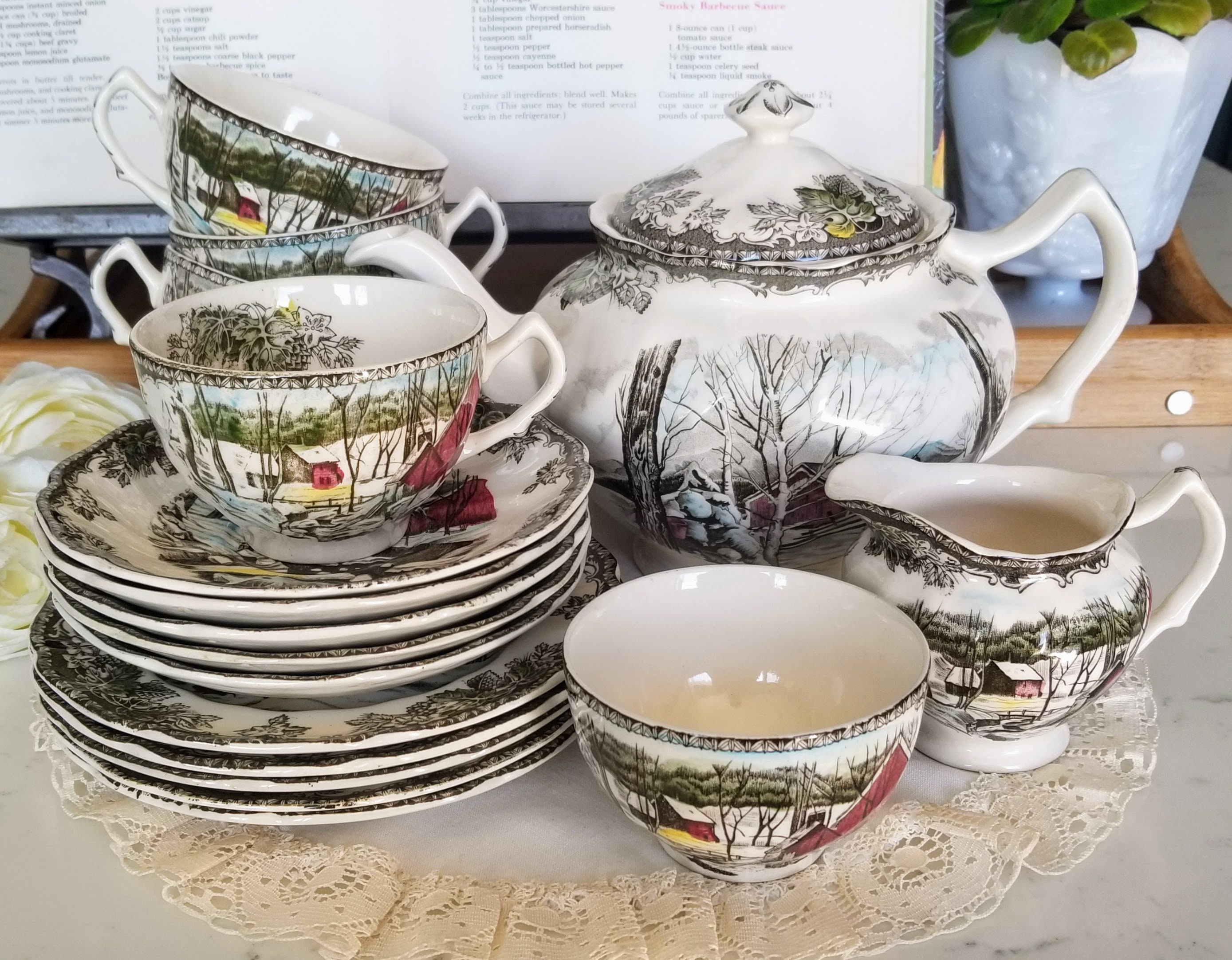This indoor photograph showcases a vintage Currier and Ives-style china set, meticulously arranged on a white lace doily placed atop a white marble surface. At the center of the display is an opened plaque or book with unreadable text, lending an air of antiquity to the scene. Dominating the left side, a stack of four to five plates is crowned by a similar stack of saucers, with a single coffee cup perched on top. Nearby, three teacups are stacked together. Central to the image, a small bowl sits prominently in front of a cream jug. Both the bowl and the creamer feature a picturesque snowy countryside landscape. To the right, a teapot, adorned with the same winter scene, stands with its handle facing right, matching the creamer’s orientation. All pieces of the set, including the teapot and cream jug, boast the detailed Currier and Ives print. Tucked slightly behind the tableware, a printed menu adds depth to the backdrop while a plant in a white glass vase peeks out from the upper right, completing this timeless composition.